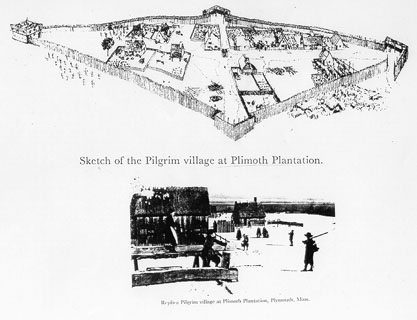This black and white illustration, titled "Sketch of the Pilgrim Village at Plymouth Plantation," presents a detailed isometric view of the historical settlement. Encircled by a wooden fence with entry breaks, the village showcases a combination of structures and open areas, suggestive of farmland for crop cultivation. Prominently, a bridge is depicted at the bottom end of the village, while a building, possibly a barn or a house, is noticeable in the left-hand corner. The presence of a man walking with a stick, along with other figures in long coats, hints at a winter setting with no visible roads or paths. Below this intricate sketch, a photograph further illustrates the village's bygone era, featuring old farm buildings and a house, possibly a school, with people—one potentially a child—outside. The image evokes a sense of historical coldness, possibly due to the snow-covered ground.